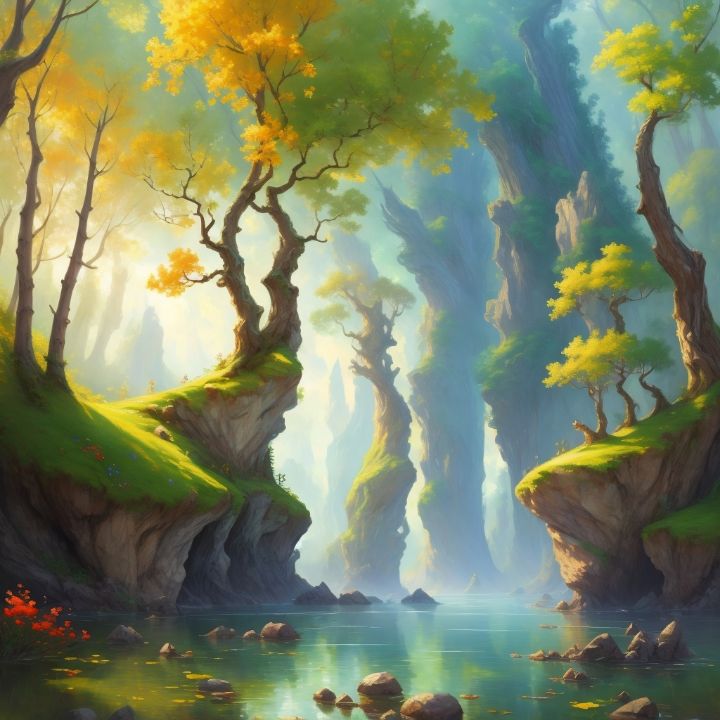The image depicts a captivating CGI animated lakeside forest scene bathed in warm, natural sunlight that pours through, giving the entire landscape a glowing, classy ambiance. From the perspective of standing in the clear, bluish-green lake, the scenery extends into hills and grassy areas dotted with an array of tall trees whose leaves vary in color from light green to vibrant yellow and orange. Some of the trees, sparsely leafed along their trunks but boasting dense clusters of foliage at their tops, rise impressively high. Scattered rocks populate the foreground of the lake, and a striking red plant juts out on the left, adding a splash of color. The background seamlessly continues this pattern of elevated land and trees, with branches softly fading into the distance. The combination of natural elements, including water, rocks, and towering trees, creates a serene and inspiring atmosphere.